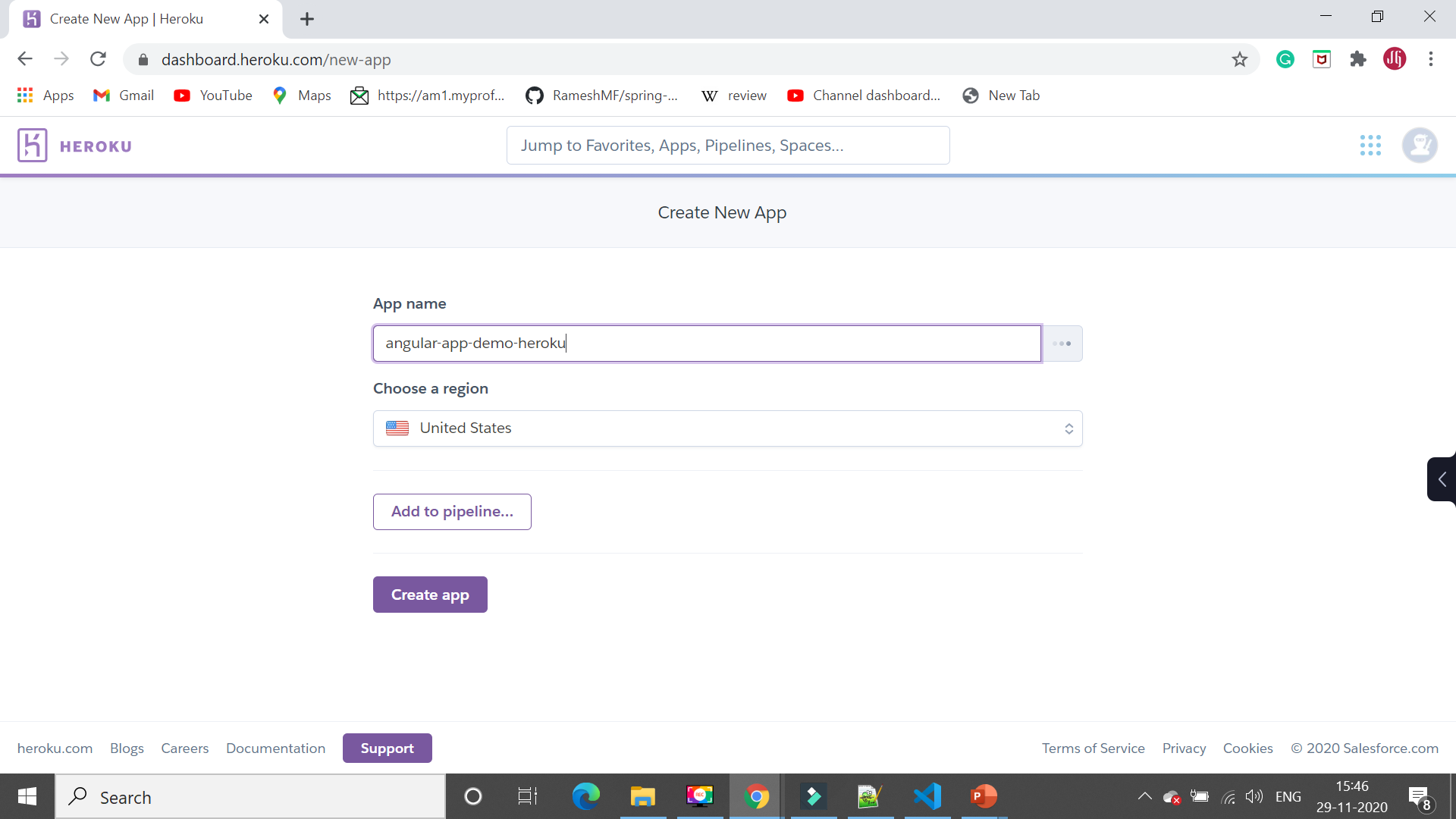This detailed screenshot captures a Chrome browser window focused on the Heroku platform, specifically the "Create New App" page. The browser's address bar indicates "dashboard.heroku.com" as the URL. Below the address bar, a bookmarks toolbar is visible, featuring shortcuts to various websites including Apps, Gmail, YouTube, Maps, Wikipedia, and another instance of YouTube, among other sites. An additional browser tab is open besides the Heroku tab.

The web page prominently displays the title "Create New App." The main section of the page contains a text field labeled "Name App," filled in with "angular-app-demo-heroku." Below, there is a section labeled "Choose a Region," featuring a drop-down menu currently set to "United States," accompanied by the U.S. flag. Further down, there is an "Add to Pipeline" button, followed by a purple "Create App" button. The background of the webpage is predominantly white.

At the bottom, the footer includes a purple "Support" button on the right. To its left are links to "Documentation," "Careers," "Blogs," and "Heroku.com." On the far right side of the footer, there are links to "Terms of Service," "Privacy," "Cookies," and a "2020 Salesforce.com" copyright note. A singular black tab is also visible on the center-right edge of the screenshot.

To the right of the address bar, there are four icons: the first resembles a timer with a green background, the second is a McAfee shield symbolizing a website virus scanner, the third is a puzzle piece, and the fourth is a red circle featuring the letters "D" and "H."